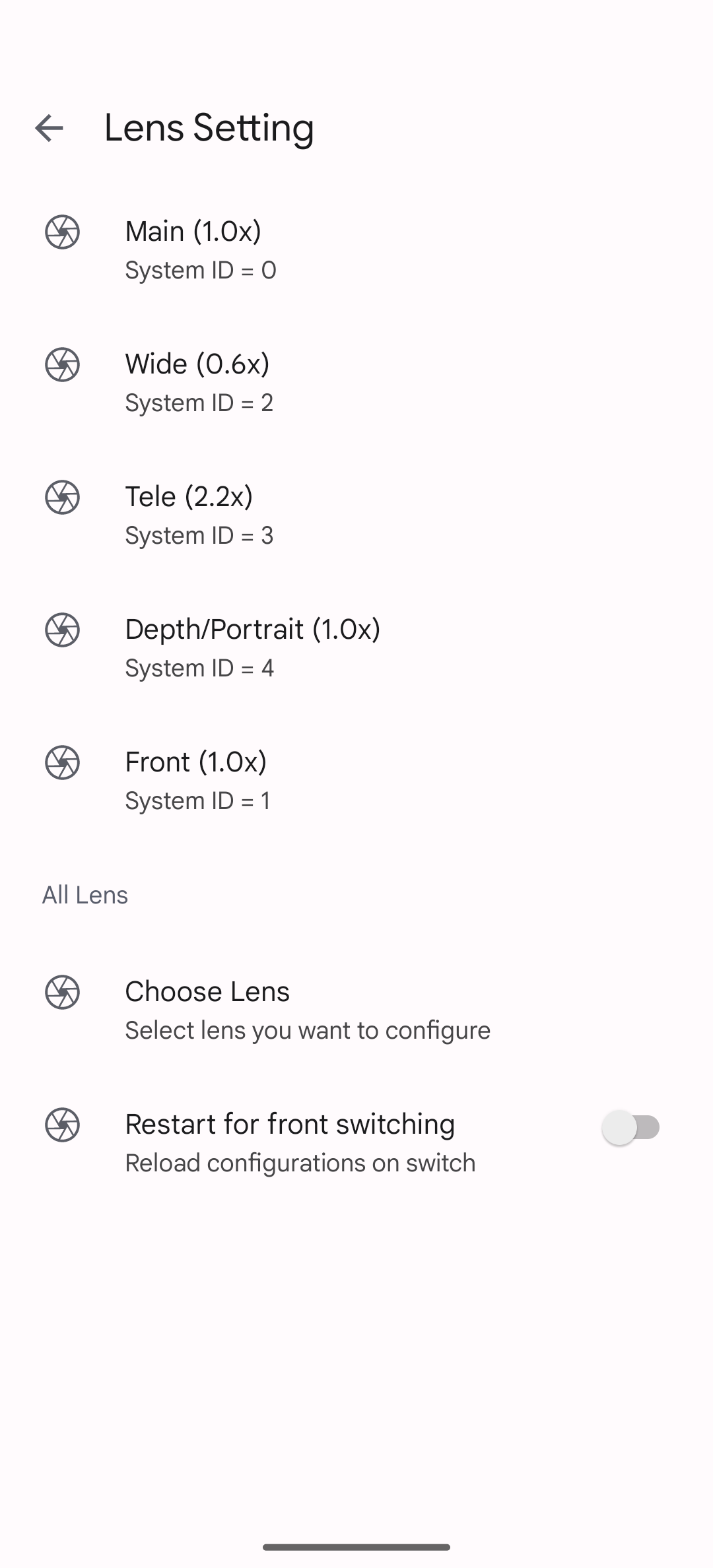The image appears to be from a settings menu on a webpage, presented against a white backdrop with all writing in black. In the upper left-hand corner, there is an outlined black arrow pointing left, next to the text "Lens Setting."

Directly beneath this, the page contains several sections, each marked by a distinct black and white circular icon resembling a beach ball. Here is a detailed breakdown:

1. **Main Lens:**
   - Icon: Black circle with a white circle rimmed in black and a black dot at the center with six black lines radiating from it.
   - Label: "Main (1.0x)"
   - System ID: "=" 0

2. **Wide Lens:**
   - Icon: Similar to the main icon.
   - Label: "Wide (1.0x 0.6x)"
   - System ID: "=" 2

3. **Tele Lens:**
   - Icon: Similar to the main icon.
   - Label: "T-E-L-E (2.2x)"
   - System ID: "=" 3

4. **Depth/Portrait Lens:**
   - Icon: Similar to the main icon.
   - Label: "Depth/Portrait (1.0x)"
   - System ID: "=" 4

5. **Front Lens:**
   - Icon: Similar to the main icon.
   - Label: "Front (1.0x)"
   - System ID: "=" 1

In the next section, we have:

- **All Lens:**
  - Label: "Choose Lens" with a subsequent instruction to "Select Lens You Want to Configure."
  - An option titled "Restart for Front Switching" with the note "Reload Configurations on Switch."
  - A gray tab containing a black ball on the left-hand side.

Finally, in the center of the page, there is a small horizontal black line.

This configuration seemingly allows the user to select different lenses and adjust settings, with an emphasis on the specifics for each type, including their system IDs and magnification values.